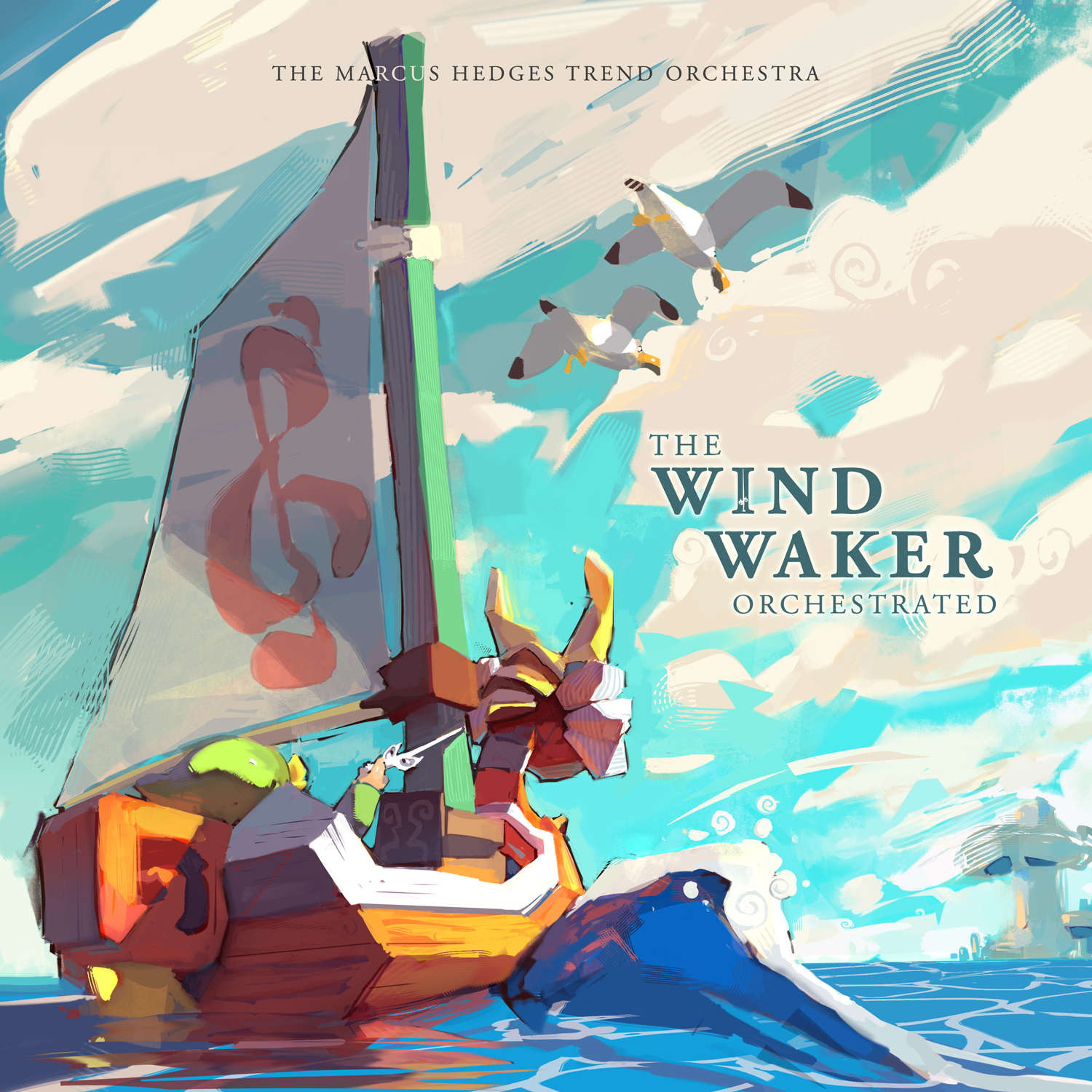The album cover features a cartoon-style, yet realistic painting of a wooden boat reminiscent of a Viking longship, complete with a dragon head at the prow and two horns. The boat, adorned with a green mast and a white sail, proudly displays a large pink musical symbol at the center of the sail. Inside the boat, the green head and shirt of a person holding a forward-pointing sword can be just barely seen. The vessel traverses blue, bubbly ocean waves while two seagulls soar in the cloudy sky above. The album title, "The Wind Waker Orchestrated," is emblazoned in the middle right section of the image, and the top of the image bears the name "The Marcus Hedges Trend Orchestra."